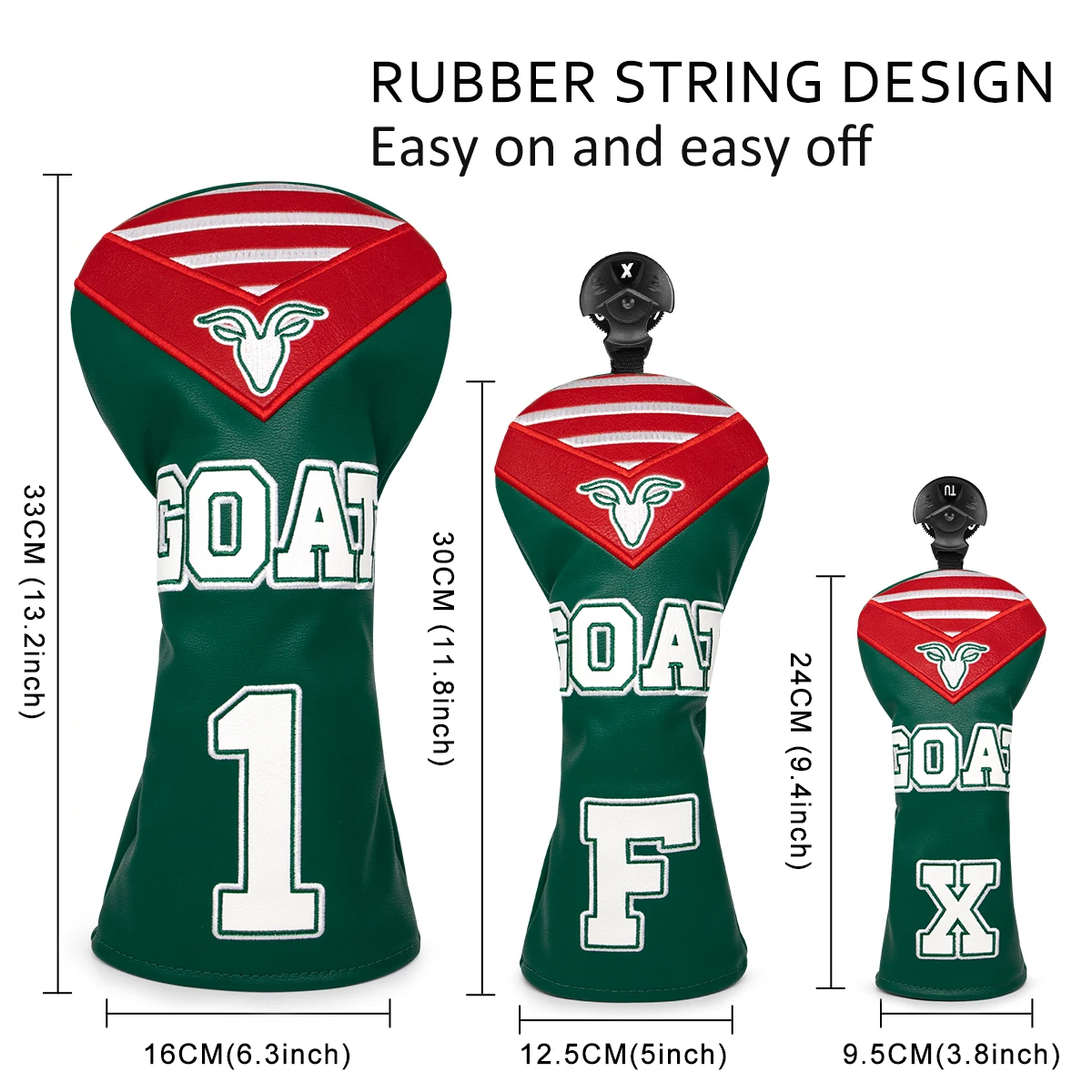This image is an advertisement depicting three bottle-shaped objects of varying sizes, each outlined against a white background. At the top, the title reads "Rubber String Design Easy On and Easy Off" in bold black lettering. The objects, each resembling a bottle, have distinctive red tops adorned with illustrations suggestive of a goat's head and horns. The main bodies of the objects are dark in color, possibly black or dark green, featuring the word "GOAT" prominently in white text. Each object is marked distinctly: the left one says "GOAT 1," the middle one says "GOAT F," and the right one says "GOAT X." Their dimensions are clearly measured, with one object's height noted as 13 inches, another as 11.8 inches, and the smallest as 9.4 inches. The design suggests these items might be easy to cover and uncover, hinting at a functional use, though their exact purpose remains unclear.